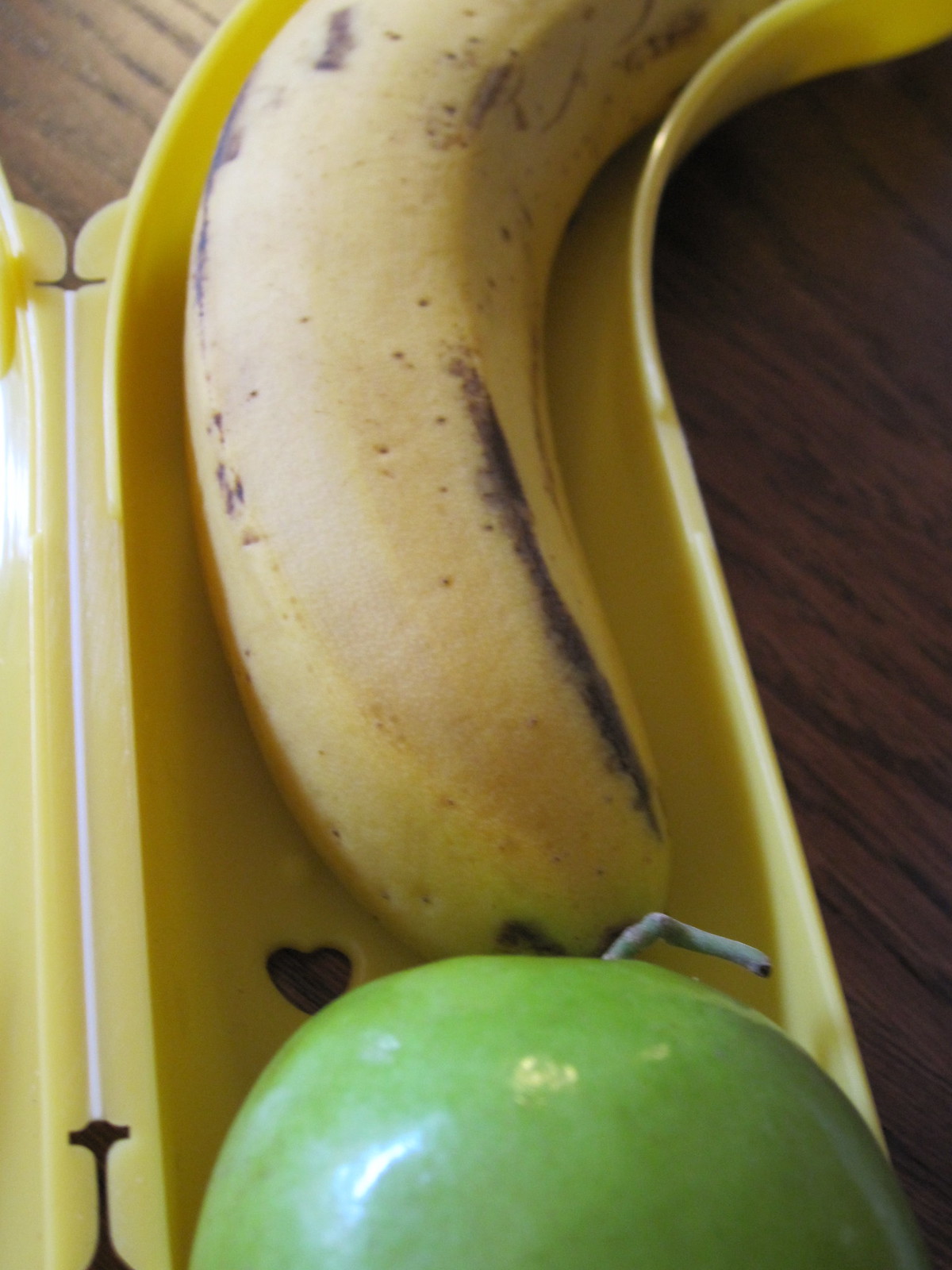The image features an extreme close-up of a yellow banana and a green apple on a brownish table. The background is faintly visible, giving a sense of the setting. The banana is laid into a yellow, container-like object that appears open, taking the same curved shape as the banana. Notably, this container has a visible heart-shaped hole on the left side. The banana itself occupies the lower two-thirds of the container and showcases a mix of yellow with some brown stripes. In the lower portion of the picture is the top half of a likely green apple, which appears exceptionally shiny—potentially due to a camera flash or overhead lighting. The apple also has a small, greenish-brown stem. The composition draws attention to the textures and shapes of the everyday fruits, creating an interesting visual contrast.